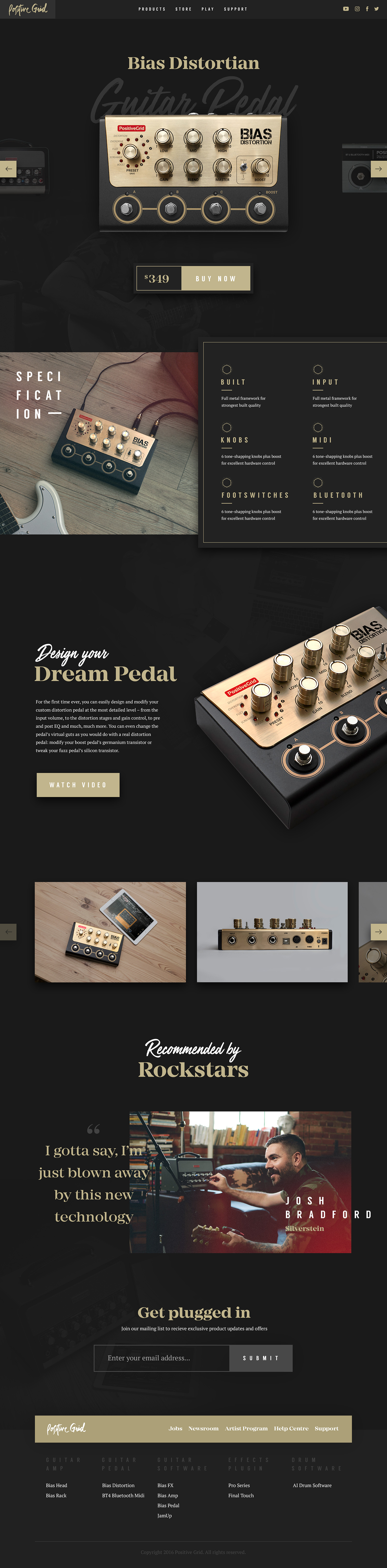This web page from a company specializing in sound mixing equipment features the "Bias Distortion" device prominently at the top. Below this title, a photograph showcases the electronic device with a luxurious golden-colored panel adorned with 8 round knobs. The lower section of this panel transitions into a sleek black surface with 4 additional knobs, each encircled in gold and interlinked by a horizontal line at the midpoint. Another photograph captures the same device positioned on the floor, now equipped with 3 cables extending from it. Accompanying this image is a black panel filled with small white text detailing the various specifications and features of the product. Further down, yet another image presents an isometric view of the device, giving a comprehensive visual perspective. Adjacent to this, bold text invites users to "Design Your Dream Pedal," while a tagline at the bottom affirms its endorsement - "Recommended by Rock Stars."